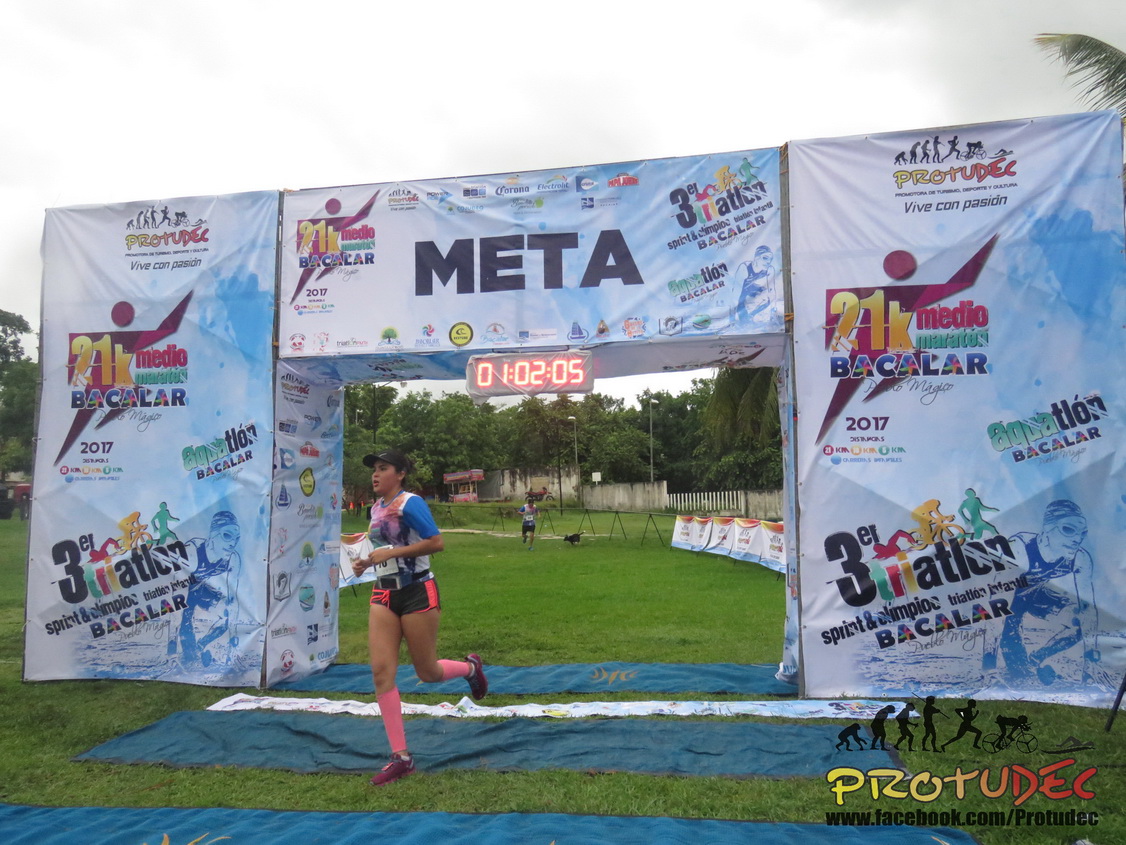The photograph captures a runner crossing the finish line of an outdoor race or marathon on a cloudy day with a white, overcast sky. The finish line is framed by a blue, square archway labeled "META," and features a digital clock displaying a time of one hour, two minutes, and five seconds. The runner, wearing a black baseball cap, pink socks, and a blue shirt, is captured in mid-stride on green grass, with scattered tarps visible in the background. Additional details include a faint appearance of another runner and a dog behind the archway, as well as surrounding fences and a house. At the bottom of the photo, there is text with the URL and logo for Produtech, which shows the evolution from a primate to a cyclist.